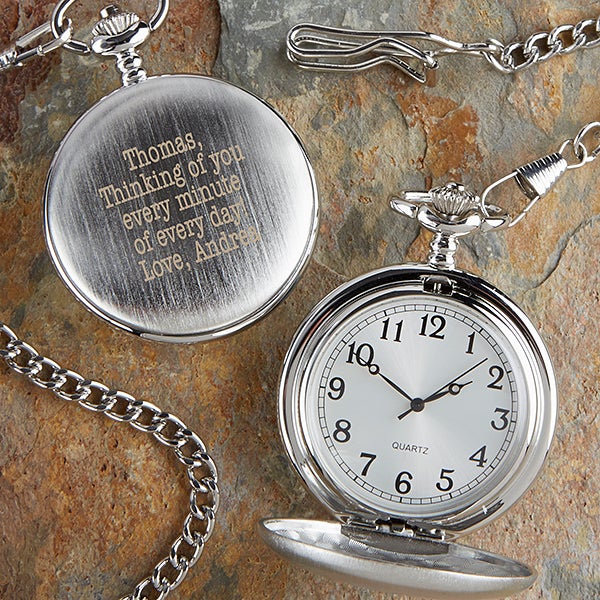In this detailed photograph, two silver pocket watches rest on a rugged, multi-colored stone surface, blending shades of gray, brown, and reddish-orange. The watch on the right is open, revealing a classic clock face with black numerals, hour, minute, and second hands against a white background. This exquisite timepiece, crafted from stainless steel, features an ornate clasp at the top, from which a silver chain elegantly drapes, partially exiting and re-entering the frame. The open watch displays the time at precisely 1:50.

The watch on the left is closed, showcasing a heartfelt engraving on its exterior, inscribed in yellow lettering: "Thomas, thinking of you every minute of every day. Love, Andrea." Both watches are seemingly identical, offering a visual exploration of their two facets – one open and functional, the other closed and intimate. The presence of the chains and clasps suggests both practicality and sentimentality, symbolizing the connection between time and personal memories.